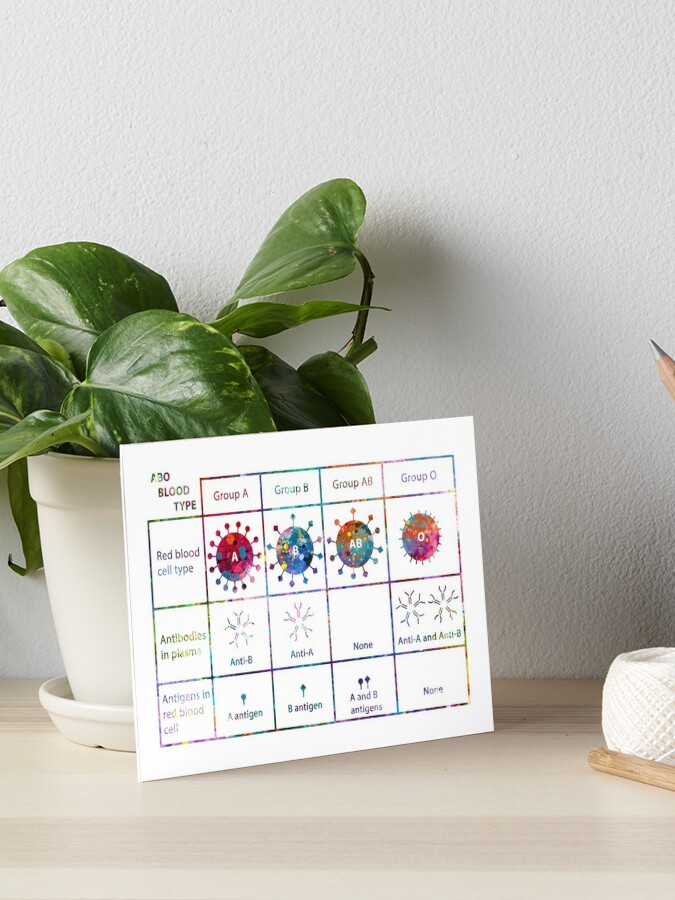The photograph depicts a detailed blood type chart leaning against a white flower pot with lush green leaves sprouting from it. The chart, which has a grid pattern, consists of four columns and three rows. The columns categorize the blood types into group A, group B, group AB, and group O, with corresponding symbols below each, including a sun-like representation of red blood cells. The rows on the left are labeled "red blood cell type," "antibodies in plasma," and "antigens in red blood cell."

In the upper left corner of the chart, the text "number 30 blood type" is visible. The second row has symbols like small Y's and circles to depict the presence of antibodies, with group AB showing none and group O having two. Anti-A and anti-B are specified under respective blood groups, with anti-B under group A and anti-A under group B. 

The setting includes a light wooden surface on which a pencil tip and a spool of white thread are visible to the right of the chart. The background features a textured wall painted in a white or slightly off-white color.